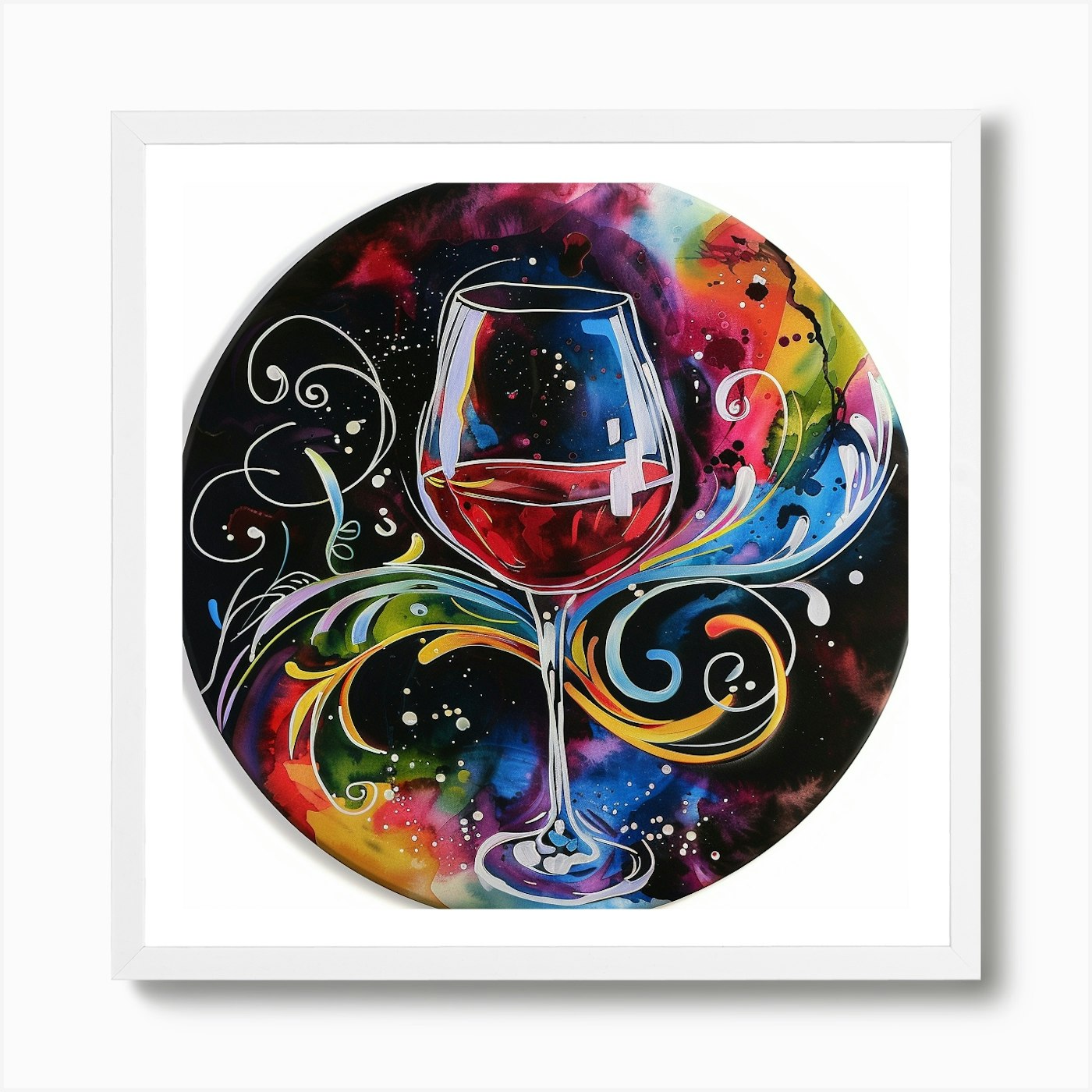Hanging on a white wall, this framed artwork features an intricately detailed painting of a wine glass filled with red wine. Encased in a white mat and slightly off-white frame, the central image is circular, yet cropped at the top, bottom, left, and right to fit the frame. The glass appears hand-blown, with a wavy rim adding a touch of craftsmanship. The backdrop is a deep, starry black, giving a cosmic vibe. Surrounding the wine glass are abstract, feathery designs with vibrant swirls and splashes of color—yellow, blue, gray, red, green, and orange—creating a dynamic, nebula-like effect. The top of the image features more vivid colors, adding to the sense of a swirling, colorful galaxy. Amidst this explosion of color, random white dots and patches contribute to the impression of a star-filled space, making the wine glass appear as if it floats in an abstract, cosmic explosion of color.